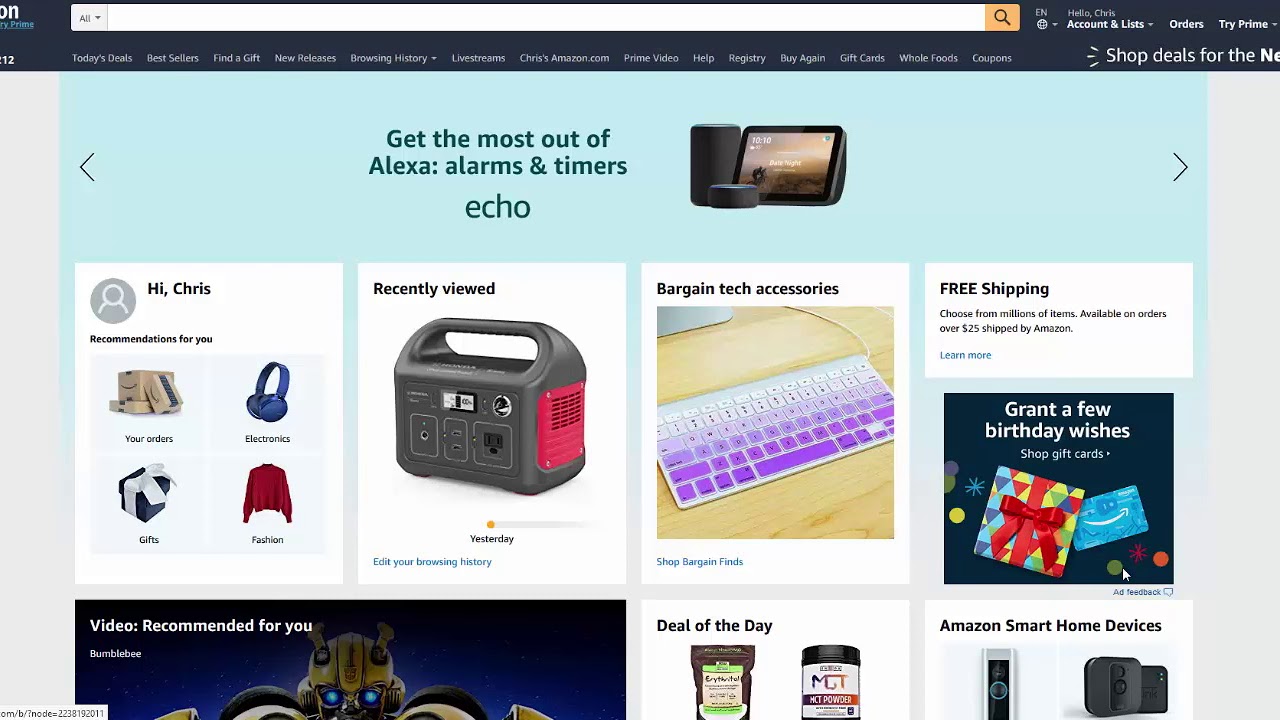The landing page on Amazon.com presents Chris’s personalized profile with a variety of features. At the top, the familiar Amazon search bar is prominently displayed, with a dropdown menu on the left side. To the right of the search bar, a welcome message, “Hello, Chris,” is shown, alongside options for "Accounts & Lists," "Orders," and "Try Prime." 

Following this header, a navigation bar provides quick access to frequently used sections, including "Today's Deals," "Best Sellers," "Find a Gift," "New Releases," "Browsing History," "Live Streams," "Chris's Amazon.com," "Prime Video," "Shop," "Registry," "Buy Again," "Gift Cards," "Whole Foods," and "Coupons." Below this navigation bar, on a light blue background with black text, it reads, “Get the Most out of Alexa: Alarms and Timers, Echo,” flanked by forward and back arrows for additional content browsing.

In the main content area, various white boxes display personalized information and suggestions. The first box greets Chris and shows recommendations tailored to him, including categories such as "Your Orders," "Electronics," "Gifts," and "Fashion." Another box titled "Recently Viewed" features an item that appears to be either a radio or a generator. The "Bargain Tech Accessories" section highlights a vibrant purple external keyboard set on a light blonde wood desk. 

Further down, another box offers "Video Recommendations for You," situated next to the "Deal of the Day" and "Amazon Smart Home Devices" sections, thus providing a comprehensive user-focused experience tailored to Chris’s interests and browsing history.